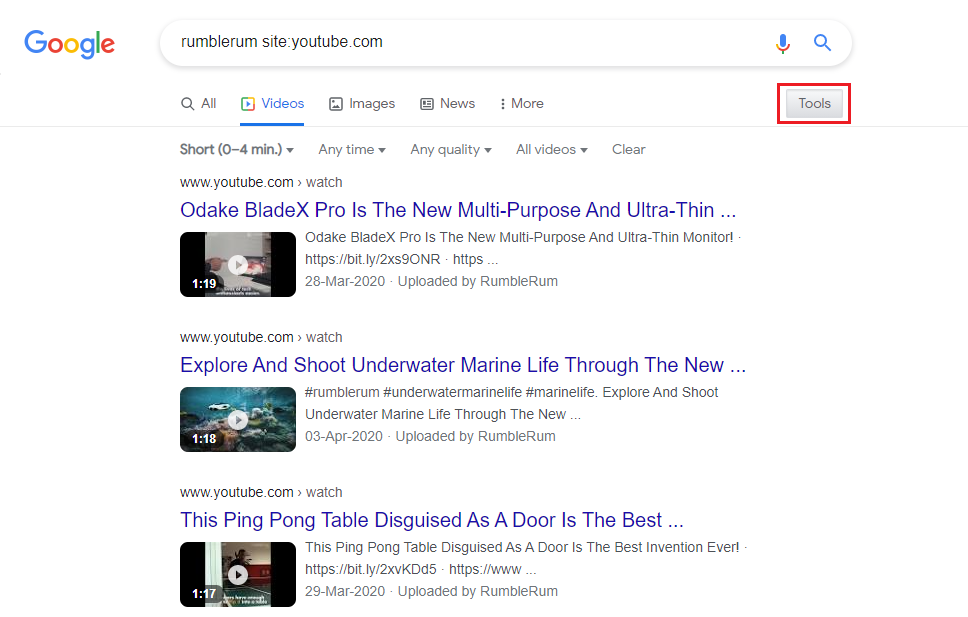Screenshot of a Laptop Displaying a Google Search Results Web Page

In the upper left corner of the screenshot, the Google logo is prominently featured with its characteristic multicolored letters: a blue “G”, red “O”, yellow “O”, light blue “G”, green “L”, and red “E”. The search bar at the center of the page contains the query: "rumble, rum, site:youtube.com". To the right of the search bar, there are three icons in succession: a speaker symbol, a microphone, and a magnifying glass.

Beneath the search bar, there are several filter options categorized under tabs. At the top, the “Tools” box is highlighted in red. Directly below it, a navigation bar lists categories: All, Videos, Images, News, and More. The “Videos” tab is highlighted, indicating that the search is filtered to show video results. Under the highlighted “Videos” tab, a sub-category is selected and denoted as "Short (0-4 minutes)”.

The search results feature three YouTube videos:

1. **Title**: “ODAKE Blade X Pro is the new multipurpose and ultra-thin...” 
   - **Description**: “ODAKE Blade X Pro is the new multipurpose and ultra-thin monitor.”
   - **URL**: www.youtube.com/watch
   - **Upload Date**: 28th of March, 2020
   - **Uploader**: RumbleRum
   - There is a small video icon next to the description representing a video preview.

2. **Title**: “Explore and shoot underwater marine life through the new...”
   - **Description**: Includes hashtags such as #RumbleRum, #UnderwaterMarineLife, #MarineLife
   - **URL**: www.youtube.com/watch
   - **Upload Date**: 3rd of April, 2020
   - **Uploader**: RumbleRum
   - The video thumbnail depicts an underwater scene with marine life.

3. **Title**: “This ping pong table disguised as a door is the best...”
   - **Description**: “This ping pong table disguised as a door is the best invention ever.”
   - **URL**: www.youtube.com/watch
   - **Upload Date**: 29th of March, 2020
   - There is an icon showing a ping pong table with a red and white wall in the background.

Each search result includes minimal descriptions and a thumbnail image that visually represents the content of the video.